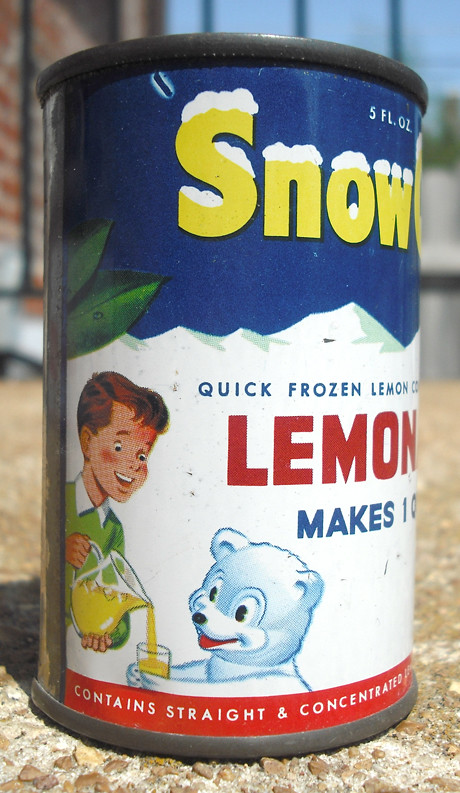This close-up photograph captures an antique-style can of lemonade concentrate, typically kept in the freezer. The can's design reflects a vintage 1950s or 1960s aesthetic. Dominating the left-hand side, the can's label features the word "Snow" in bold, yellow letters adorned with snow on top, set against a blue background. Below "Snow," the partially visible logo reads "Quick Frozen Lemon" in blue text over a white backdrop resembling snowy mountains. Towards the lower section, the word "Lemon" appears prominently in red capital letters with the phrase "Makes 10" partially cut off beneath it.

The can's top edge displays "5 FL ounces" in small white letters on a blue background, while the bottom edge bears the partially visible text "Contains straight and concentrated" in white on a red background. The can includes a charming 2D cartoon illustration: a young Caucasian boy in a green long-sleeved shirt is pouring lemonade from a clear pitcher into a glass held by a smiling polar bear, emphasizing a cheerful, nostalgic vibe. Set against a blurred background with tan and white cobblestone and distant images of a brick building and blue sky, the can is bordered at the top by a black rim and features a visible seam line extending vertically.